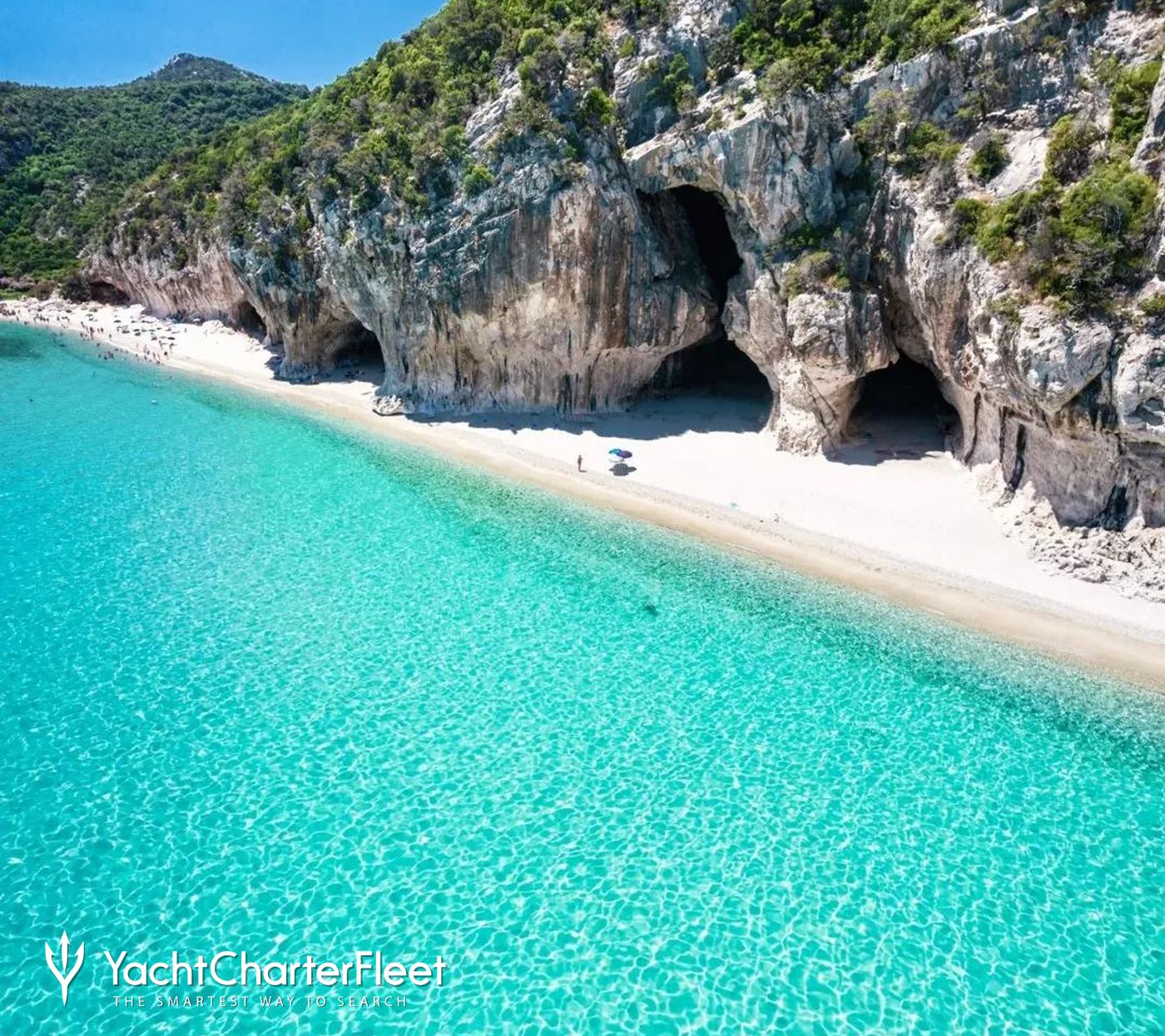The image captures a vibrant, tropical beach scene characterized by pristine, white sand gently sloping towards brilliantly blue, clear water reminiscent of the Caribbean. The water, appearing almost turquoise, displays a subtle ripple effect with white lines crisscrossing in a marble-like pattern. In the foreground, a lone person stands near the center-right, adding perspective to the scene. The beach itself is flanked by a rugged, rocky coastline with green vegetation splotched throughout the gray rock formations. These formations house at least five distinct caves, one shaped intriguingly like an hourglass. Behind the beach, a gathering of people is visible in the distance. The upper left part of the image shows a bit of blue sky coupled with mountainous rocks and some green trees. In the lower left-hand corner, white lettering spells out "Yacht Charter Fleet," accompanied by a logo resembling a stylized Y with an anchor. The entire scene is bathed in bright sunlight, emphasizing the tropical allure.